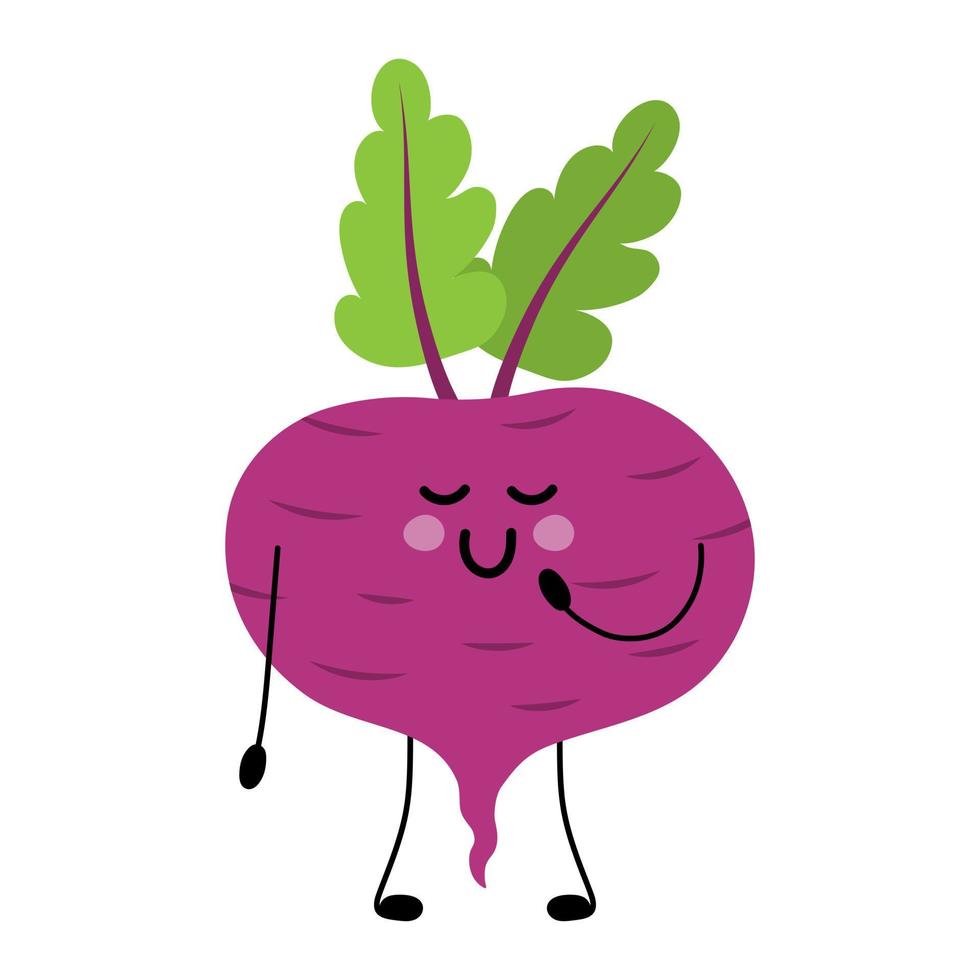The cartoon drawing features a whimsical depiction of a turnip rendered in a comic style. The turnip is purple and adorned with horizontal dark purple lines to add texture. At the top of the turnip, two antenna-like stems with bright green leaves extend upwards. The turnip has a cheerful face highlighted with rosy blush on its cheeks and closed, U-shaped eyes. It sports a big, U-shaped smile. The turnip has stick-like arms and legs, all drawn in black, with the left arm bent upward, touching the side of its face, and the right arm hanging by its side. Its feet are oval-shaped and turned inward, giving it a pigeon-toed stance. Adding to its quirky appearance, a wavy purple tail extends from its side.